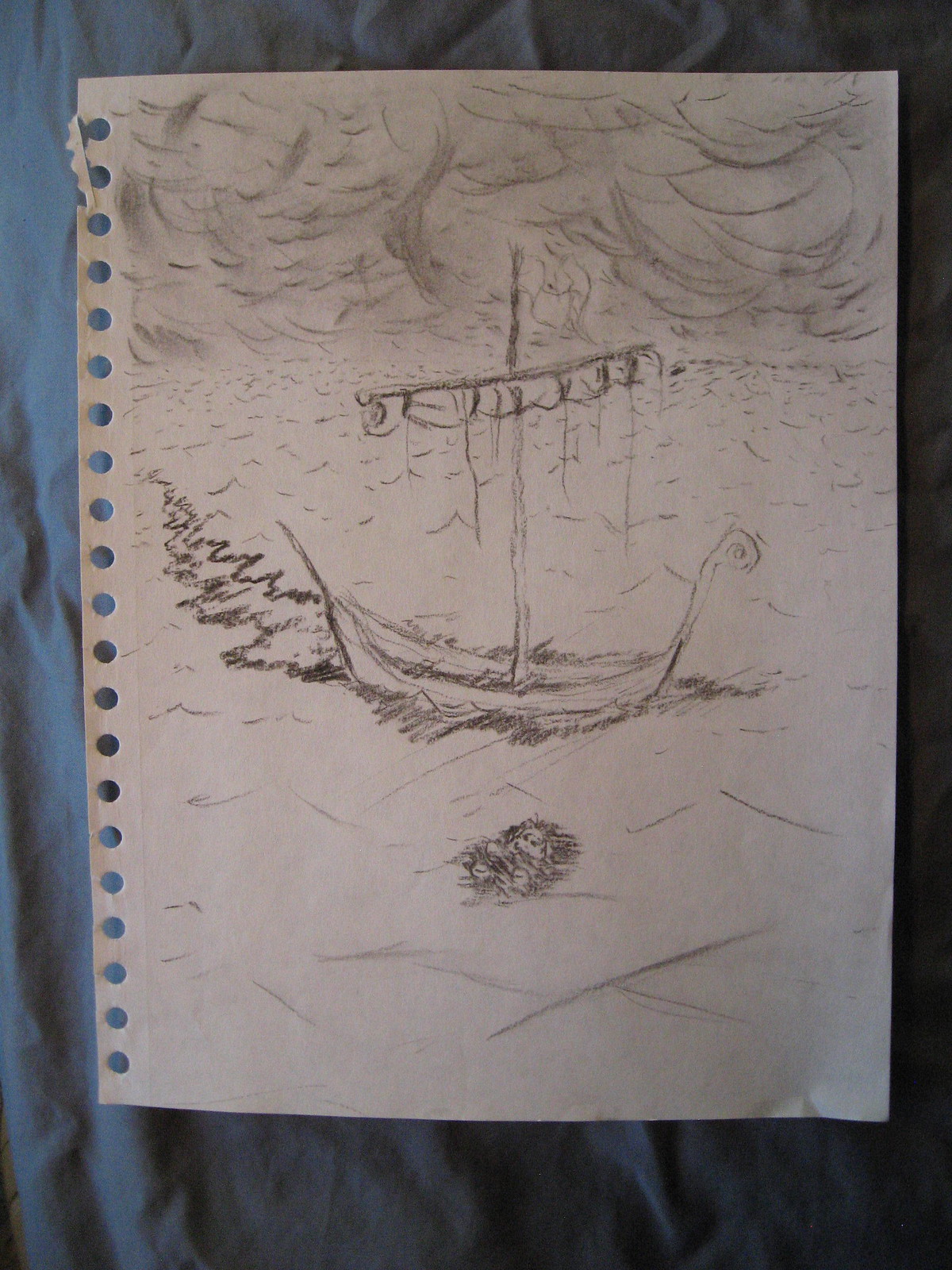A lightly sketched drawing on white paper with perforated edges is placed on a wrinkled black cloth. The artwork depicts an empty boat with a high prow and stern beached on the shore. Tidal riffles suggest the tide is coming in. The boat's sail is fully furled at the top, and the sky above appears cloudy and stormy. In the foreground, there is a vague, indeterminate figure that could be a creature or a human, though it is not clearly defined.